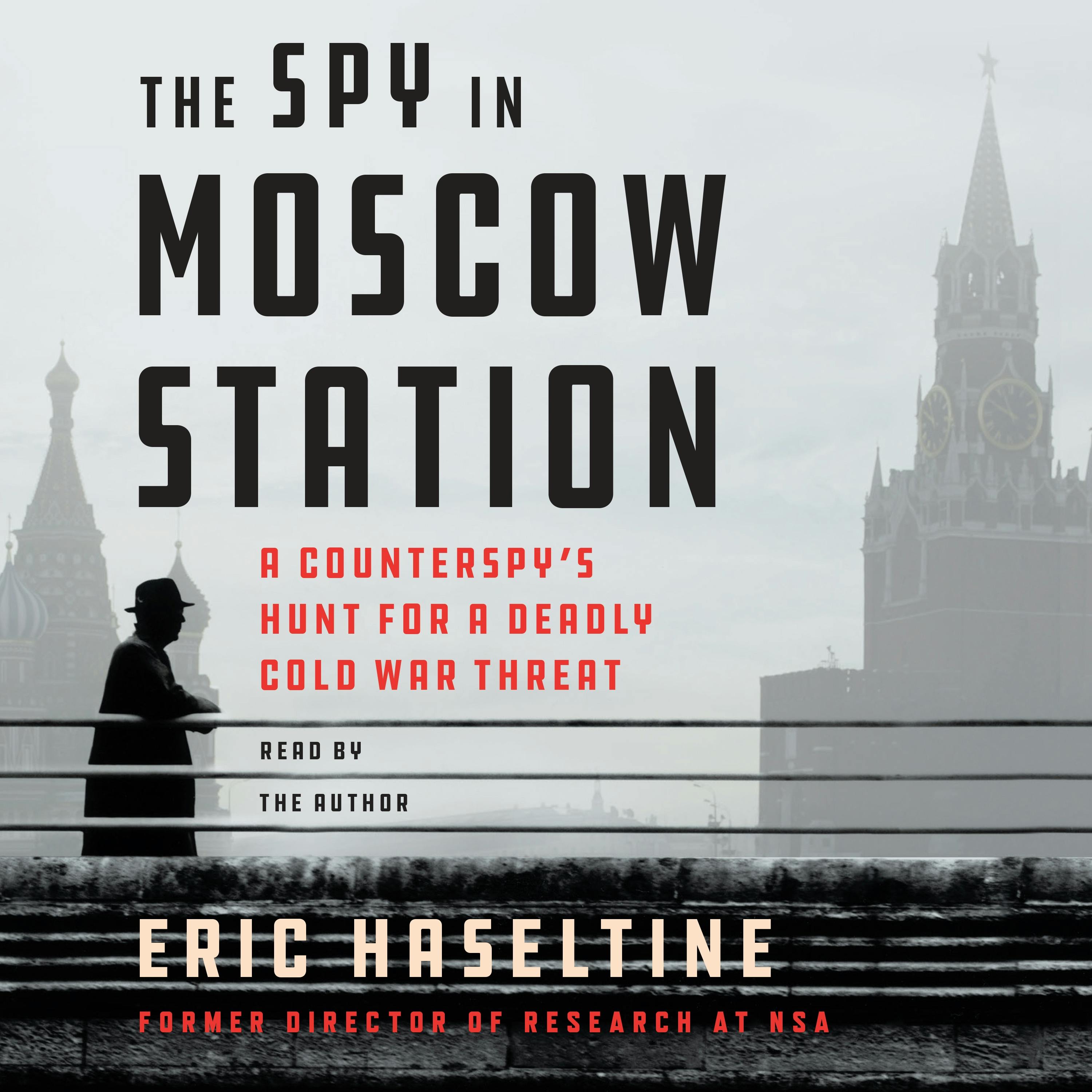This is the cover of an audiobook, presented in shades of black, white, and gray, measuring approximately 5 to 6 inches square. Dominating the top portion of the cover, slightly left of center, the title "The Spy in Moscow Station" is displayed in bold black print, followed below by the subtitle "The Counterspy's Hunt for a Deadly Cold War Threat" in smaller red print. Underneath, it states in black letters, "Read by the Author," and at the bottom in a cream color, the author's name, "Eric Haseltine," with the designation "Former Director of Research at NSA" in red below it.

The visual composition features a stone bridge at the lower section, rendered in shades of gray. The bridge includes three horizontal metal bars about an inch above its base. Leaning against these bars on the left side is the black silhouette of a man wearing a hat and a long coat. The background is largely in light gray, showcasing two prominent buildings. To the right, there's an edifice with a star-topped peak and clocks flanking its sides, suggestive of traditional Russian architecture. To the left, another structure rises, characterized by three spikes atop. The overall atmosphere is somber and cloudy, fitting the Cold War theme suggested by the title.